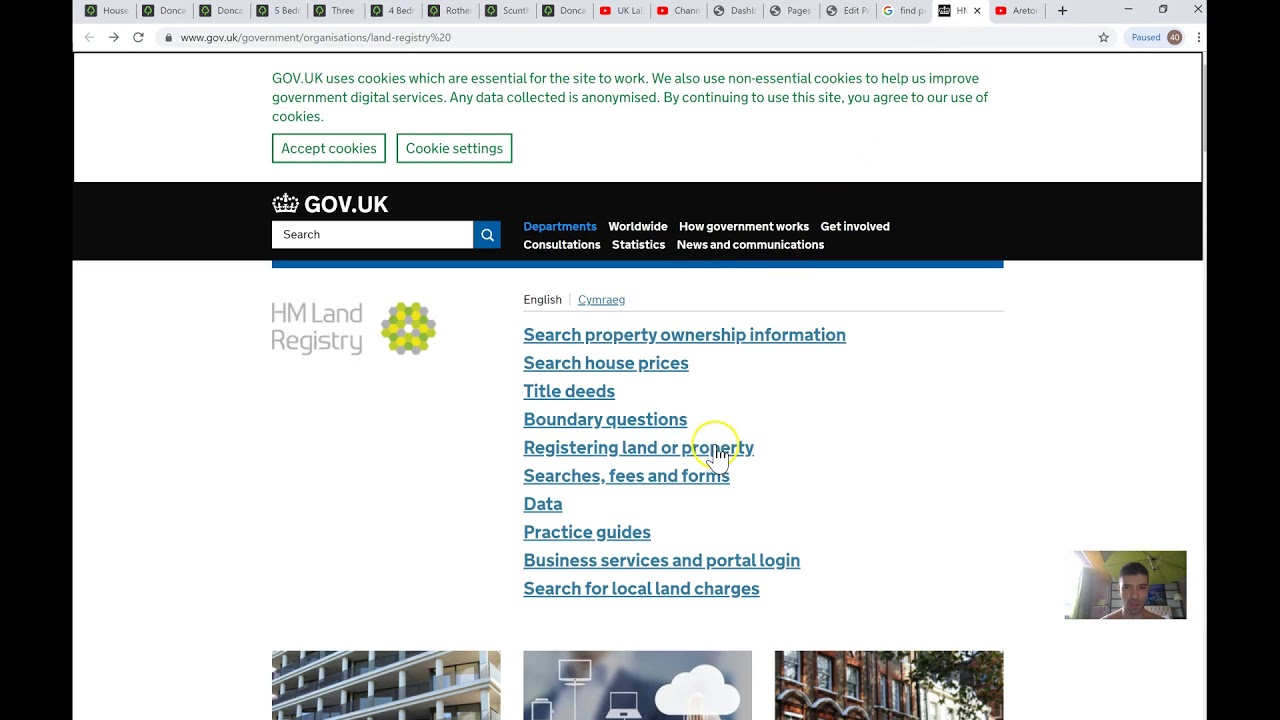The image displays a web browser with 17 tabs open, currently highlighting a webpage from the official UK government website, specifically the Land Registry section. The web address visible in the browser's address bar is www.gov.uk/government/organisations/land-registry. At the top of the webpage, there is a cookie consent banner in green font, stating, "Use cookies which are essential for the site to work." Directly below, the recognizable gov.uk header is shown, featuring a search bar. The site navigation menu includes options such as "Departments," "Consultations," "Worldwide," "Statistics," and "Get Involved."